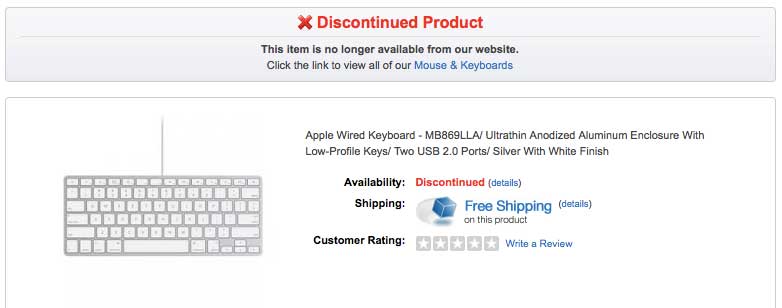The image showcases a website revealing an error message for a product that is no longer available. The website's background is predominantly white with subtle grey accents. At the very top of the page, a horizontal grey bar is prominently displayed, with the text "Discontinued Product" in bold red lettering. Beneath this, a message reads, "This item is no longer available from our website. Click the link to view all of our mouse and keyboards," with "mouse and keyboards" being a clickable hyperlink. 

Below the message is a large white box containing an image of an Apple Wired Keyboard, characterized by its sleek silver and white design. To the right of the image, detailed product information is provided, stating: "Apple Wired Keyboard MB869LL/A - Ultra Thin and Anodized Aluminum Enclosure with Low Profile Keys / Two USB 2.0 Ports - Silver with White Finish."

Further, three informational sections are listed:
1. **Availability:** Displayed in red, it states "Discontinued" with a link titled "details" in parentheses.
2. **Shipping:** Indicates "Free shipping on this product."
3. **Customer Ratings:** Notes that no ratings have been provided yet but offers an option for users to write a review.